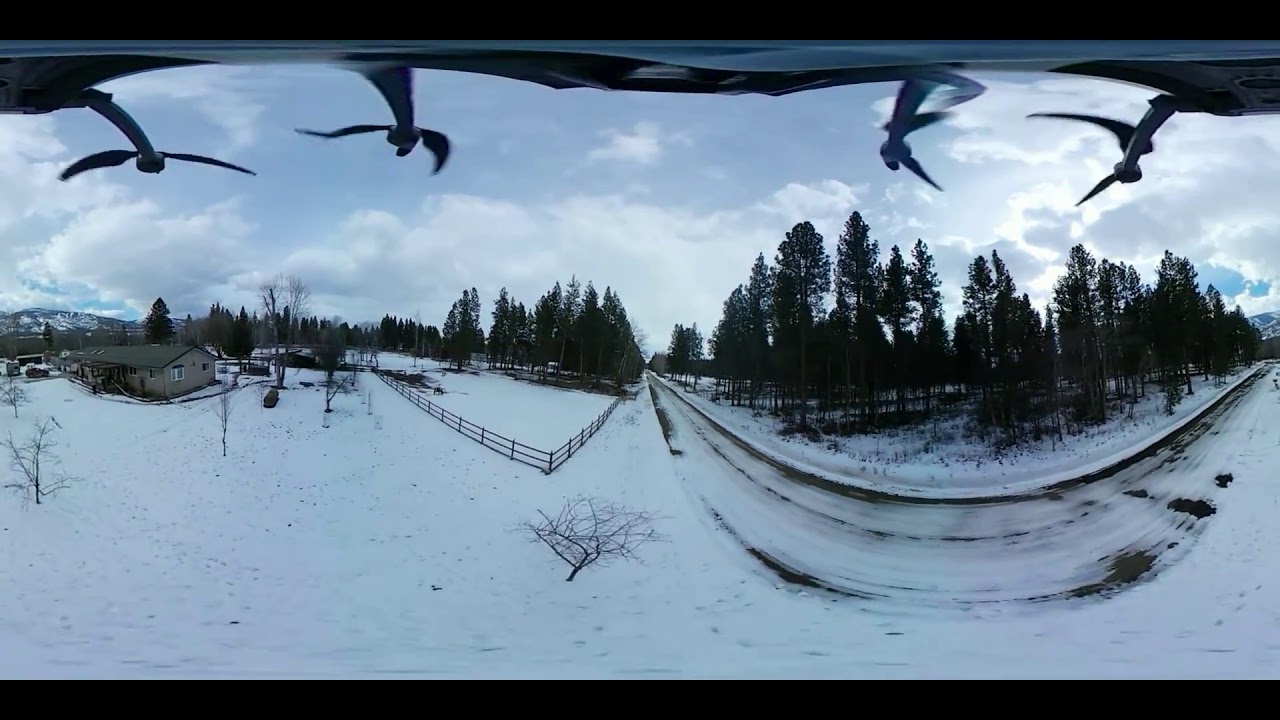This photograph captures a picturesque winter scene of snowy farmland from an aerial perspective. Dominating the landscape is a blanket of white snow stretching across the ground, intersected by a winding path that curves from the background to the foreground and back again. On the left side of the image stands a modest, one-story brown house, likely a farmhouse or ranch. Nearby, a small fence meanders through the snow, adding a rustic touch to the composition.

Evergreen trees, resembling Christmas trees, dot the landscape, their dark silhouettes contrasting against the snowy backdrop. Despite the season, they retain their foliage, contributing to the scene's festive atmosphere. In the middle of the ground, a few bare bushes and a leafless tree stand starkly against the white snow.

The sky is overcast with dark, brooding clouds, yet the sun makes a subtle appearance, peeking through the clouds on the right side of the image. This interplay of light and shadow casts a grey hue over the scene, enhancing the wintry mood.

Interestingly, the top part of the photograph reveals what appears to be propellers or pointed structures, indicating that the image was taken from a drone, providing a panoramic, bird's-eye view of this serene snowy farmland.